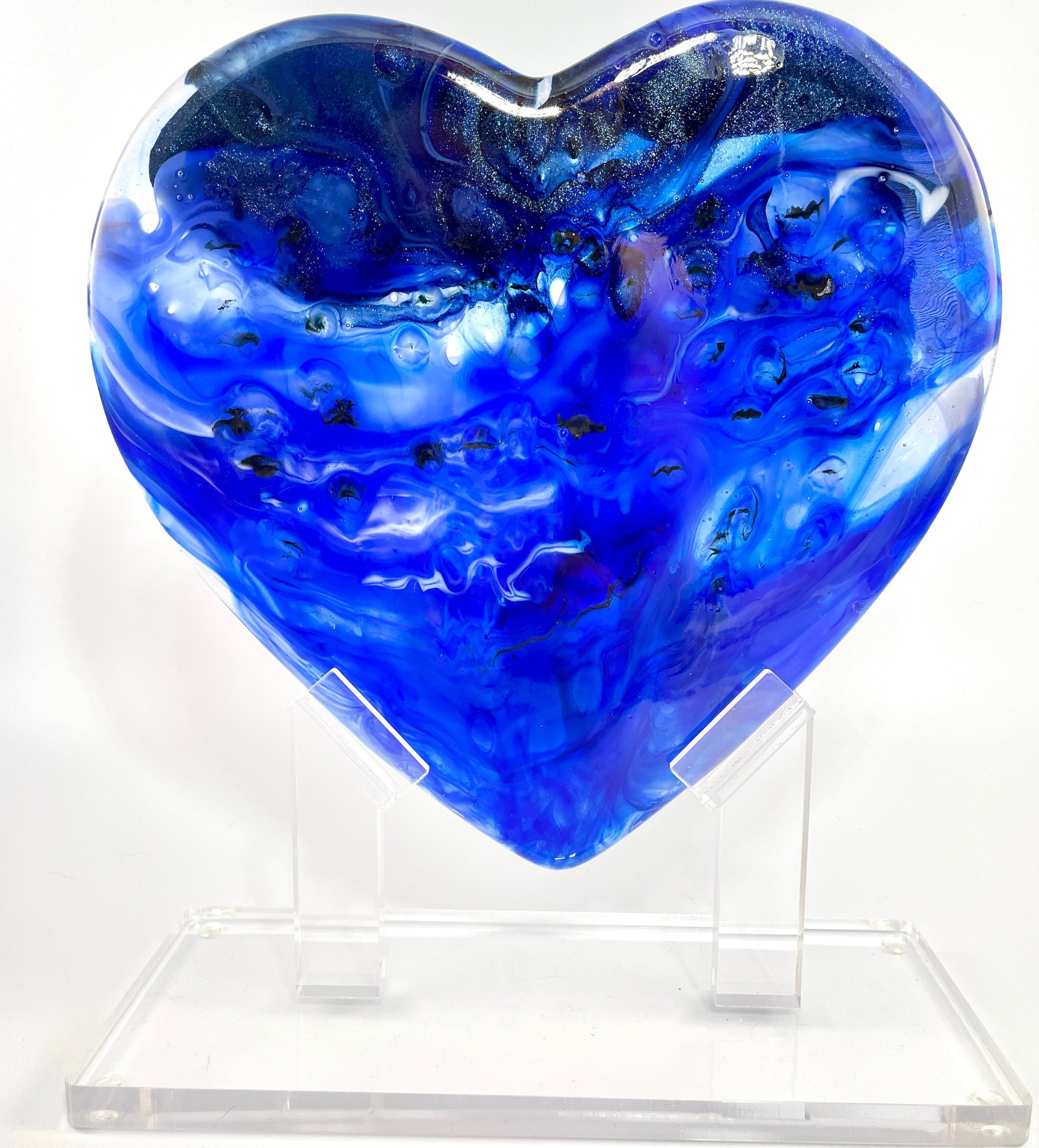This is a detailed photograph of an artistic, large blue heart sculpture, seemingly made of blown glass, mounted on a sturdy clear plastic, or possibly lucite, stand. The heart features an array of rich blue hues, from deep to light blues, intermixed with delicate swirls and bubbles, and hints of white and glitter. These details give the heart a lustrous and somewhat magical appearance. The sculpture is anchored by two transparent brackets on the stand, which make it appear as though the heart is floating. The base is a thick, clear square, providing stability and enhancing the elegant and ethereal presentation of the heart.